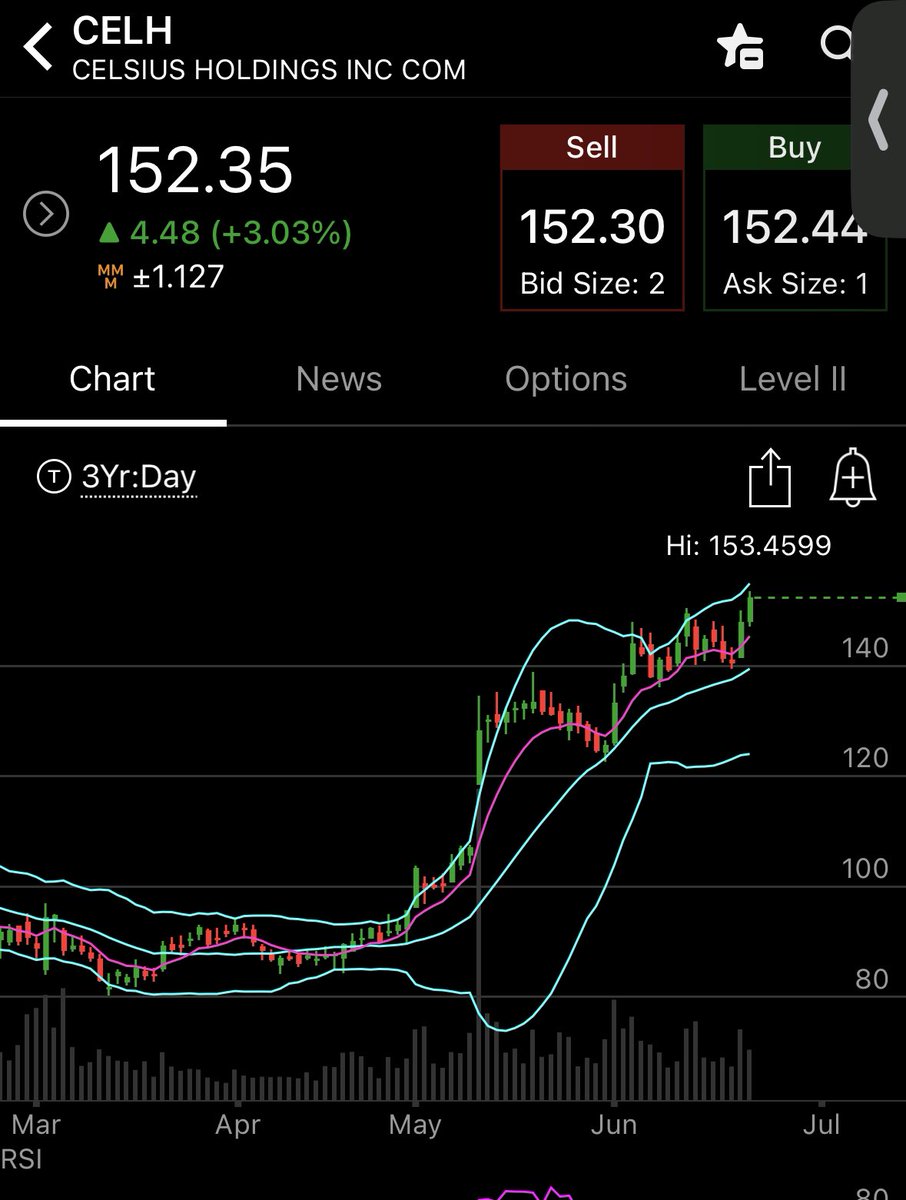**Detailed Descriptive Caption:**

The image depicts a detailed stock analysis interface against a black background, possibly sourced from a financial platform like Yahoo Finance or TradingView. The focal stock is Celsius Holdings Inc. (CELH), currently trading at $152.35. On this particular day, the stock price increased by $4.48, which translates to a gain of 3.03%. 

Two actionable buttons are visible: one for CEL trading at $152.30 and a buy button priced at $152.44. The existing bid size is two, while the ask size stands at one. Navigational tabs include options for "Chart," "News," "Options," and "Level 2," with the current focus set to "Chart."

The chart below visualizes stock performance data ranging from March through June. Notably, the stock price escalated from approximately $80 in March to roughly $90 in April and surpassed $100 in May. By mid-June, the stock peaked near $153, reaching a high of $153.4599. The chart employs red and green candlesticks to illustrate price fluctuations, supplemented by lines that likely represent moving averages or other technical indicators. 

An RSI (Relative Strength Index) panel is located at the bottom of the chart, although it's partially cut off. Additionally, a star button at the top offers a feature to bookmark or favorite the stock. This comprehensive analysis tool provides an array of data essential for detailed stock evaluation.